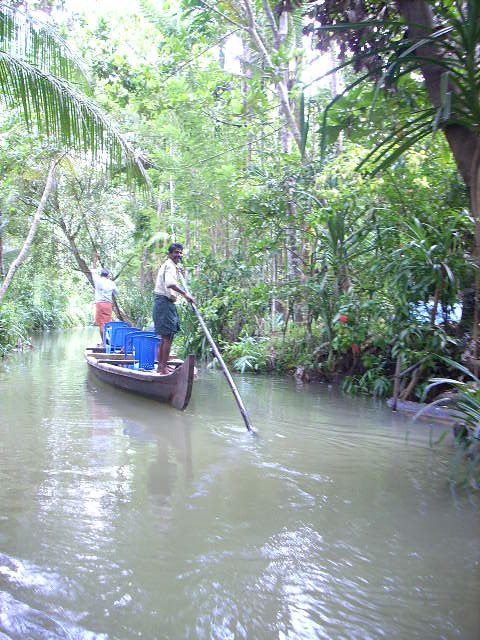In this image, a tropical jungle scene unfolds around a murky green waterway, possibly a pond or creek. The dense foliage comprises various palm leaves cascading down from both the left and the upper right sides of the frame, interspersed with tree trunks and branches. Central to the composition is a long wooden canoe, stationed slightly to the left, with two men aboard. Each man stands at opposite ends of the canoe, holding an oar or pole to steer the boat through the water. The man at the front, dressed in a light-colored shirt and gray shorts, has brown skin. Inside the canoe, amid the men and navigating tools, are blue buckets and plastic chairs, highlighting their makeshift journey through this lush, sunlit jungle environment. The water reflects sunlight, suggesting a clear, rain-free day in this verdant landscape.